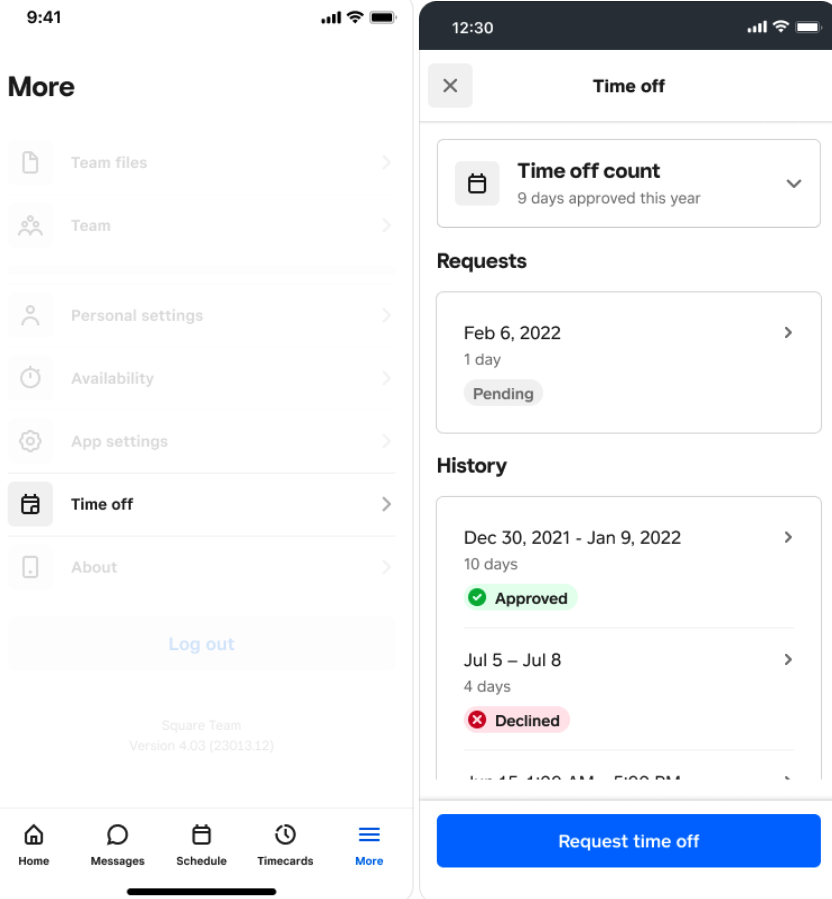This screenshot displays an employee tracking application. The interface is divided into distinct sections. On the left-hand side, there is a comprehensive menu that includes options such as "Team Files," "Team Personnel," "Personal Settings," "Availability," "App Settings," "Time Off," and "About." 

The main area on the right-hand side focuses on the "Time Off" page. Key details are prominently shown here: 
- "Time Off Count" indicates that nine days have been approved this year.
- A section for requests specifies that a time-off request was made for February 6, 2022, which is currently pending.
- The "History" section provides a detailed log of previous time-off records, including:
  - December 30, 2021, through January 9, 2022: Ten days approved.
  - July 5 through July 8: Four days declined.

At the bottom of the screen, there's a fixed navigation bar that offers quick access to "Home," "Messages," "Schedule," and "Time Cards."

Overall, this page is designed for employees to manage and request time off, view their time-off history, and navigate through essential features of the app.